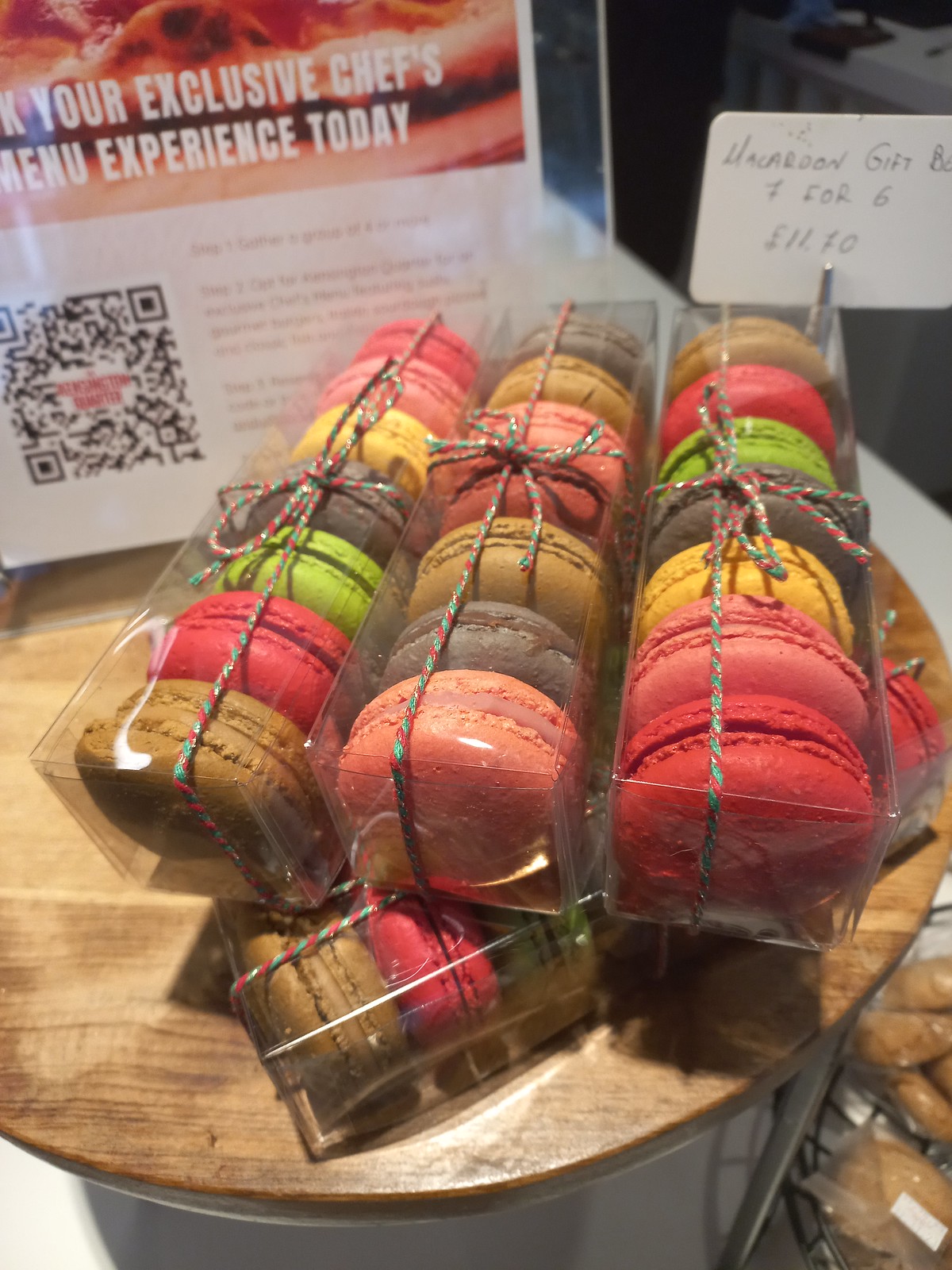This detailed color photograph captures a vibrant display of macarons, meticulously arranged in three clear plastic boxes, each tied with multi-colored yarn. The macarons, showcasing a delightful array of hues—brown, red, green, pink, yellow, and dark brown—are stacked vertically on a small, round wooden table. Beneath these boxes, more packaged macarons are partially visible. Behind the display, two signs provide context: one is handwritten, offering a "Hare Boone Gift Box 7 for $6.00," while the other, partly readable, promotes "Your exclusive chef's menu experience today." The entire scene is suggestive of an inviting shop setting, with additional details like a scannable code and imagery of food enhancing the ambiance.